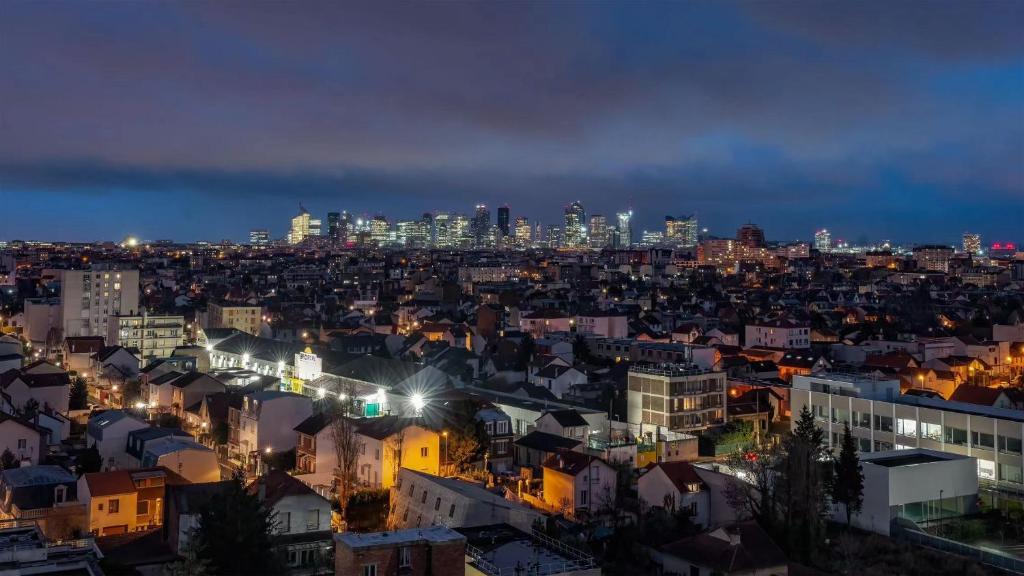This nighttime photo captures a sprawling cityscape, with a clear distinction between residential suburbs in the foreground and towering skyscrapers of the city's core in the distance, their windows illuminated brilliantly against the night sky. Dominating the left-center of the image, a very large building with bright white lights stands out among the darker, quieter homes around it, which are sparsely lit. Towards the bottom right, a long white building with a blue roof, resembling a college campus or a substantial apartment complex, features prominently, bordered by evergreen trees and a road. The sky, draped in dark gray clouds with patches revealing a dark blue hue, occupies the upper half of the frame, enhancing the nocturnal atmosphere. The photo, likely taken from an elevated vantage point such as a building, drone, or helicopter, effectively showcases the contrast between the brightly lit urban center and the more subdued residential areas, unified by the common play of various lighting—white, yellow, and orange—that punctuates the scene.